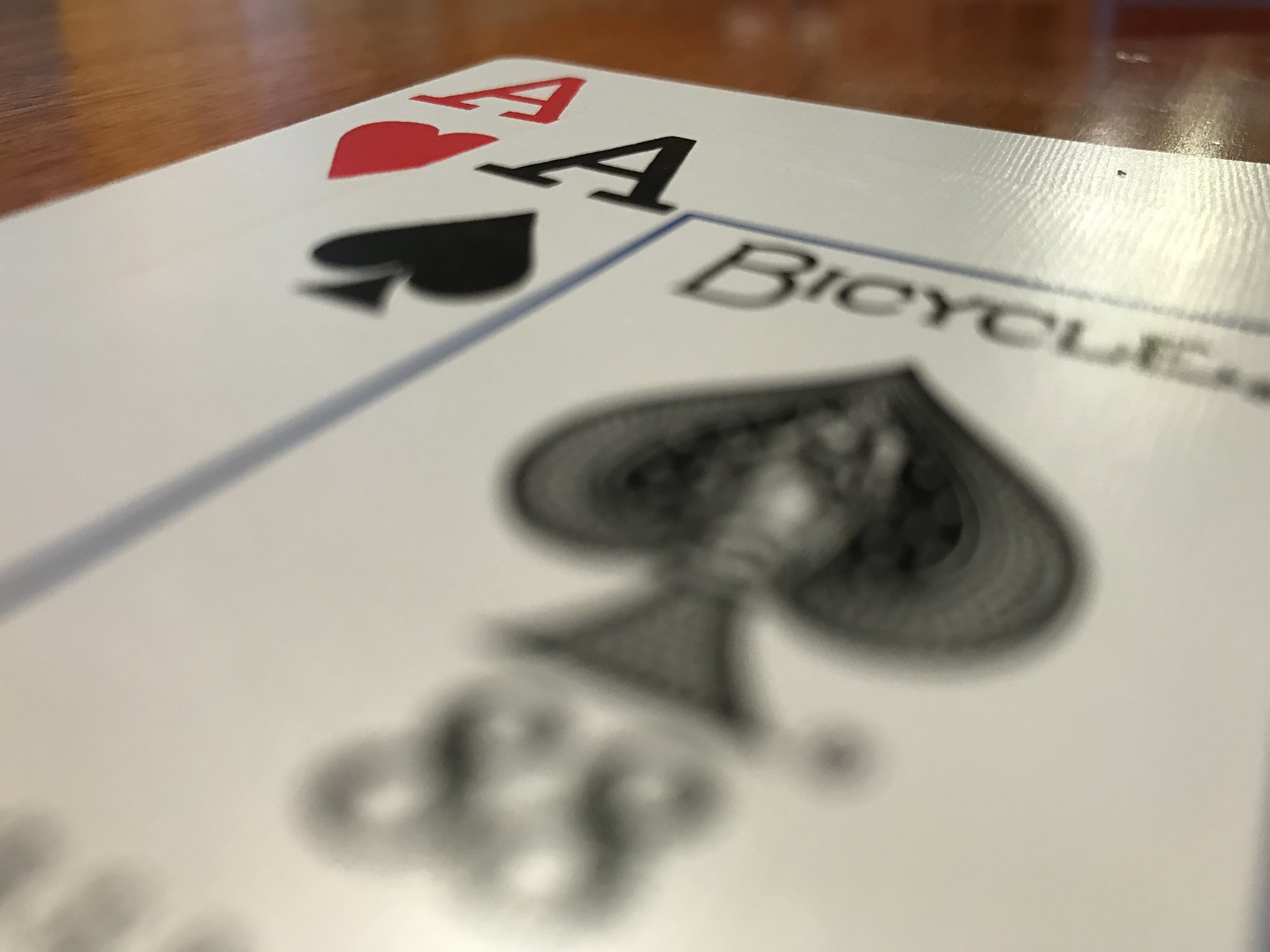The image features a close-up view of two playing cards stacked atop each other, captured at an angle to prominently display the top left corners of the cards. The top card is the Ace of Spades, while the bottom one is the Ace of Hearts. The center of the Ace of Spades card is highlighted with the word "BICYCLE" in bold, uppercase letters. Additionally, the card exhibits a large black spade symbol and the number 88, both of which appear slightly blurred, as if influenced by a tilt-shift effect. The cards rest on a surface with a wood grain texture, potentially suggesting a wooden table. The cards themselves show the wear of use and subtle textural details. The font used for the letter 'A' is a traditional serif typeface, adding a classic touch to the overall composition.